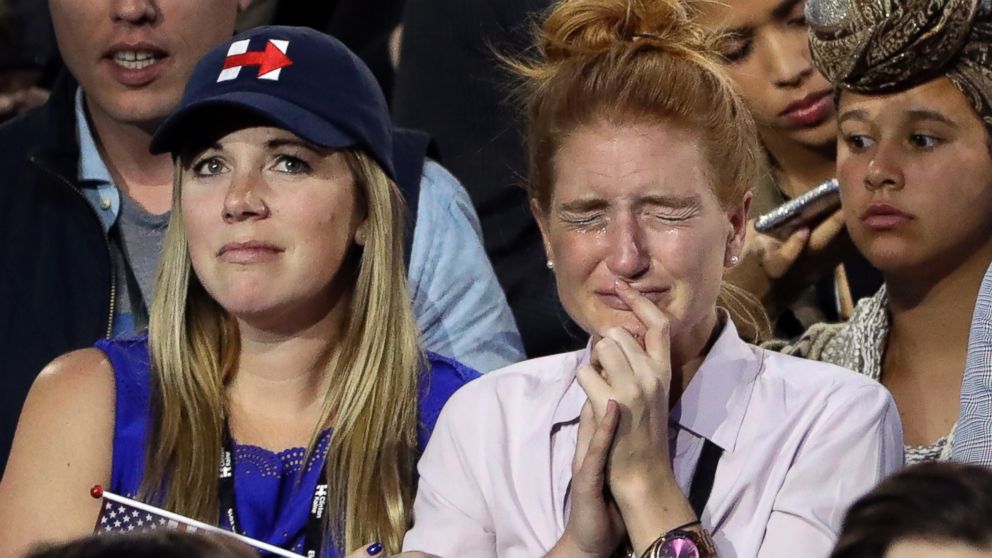The image depicts a somber scene at a Democratic political convention, featuring a small crowd of distressed individuals. At the center is a woman with long blonde hair tied back into a ponytail, wearing a blue sleeveless top and an "I'm with Hillary Clinton" baseball cap adorned with white lines and a red arrow design. She clutches an American flag and appears on the verge of tears, her nose wrinkled and right eye streaming.

To her right is another woman with blonde hair, clad in a white button-down shirt and a purple watch. She is visibly crying, her eyes shut tight, and her expression conveys deep emotion as she cups her chin with one hand. Nearby, a woman with reddish hair styled in a messy bun wears a purple collared shirt and holds a finger to her mouth, her distressed face marked by teardrops.

In the background, behind the women, a man with an open mouth stands partially visible. Additionally, one woman wearing a religious or decorative headpiece gazes off to the side, while another woman behind her looks at her phone with a concerned expression. The bottom right of the image is slightly cropped, showing just the lower corner of another man's face. The overall composition captures the raw emotion of its subjects, highlighting the poignant atmosphere at the convention.